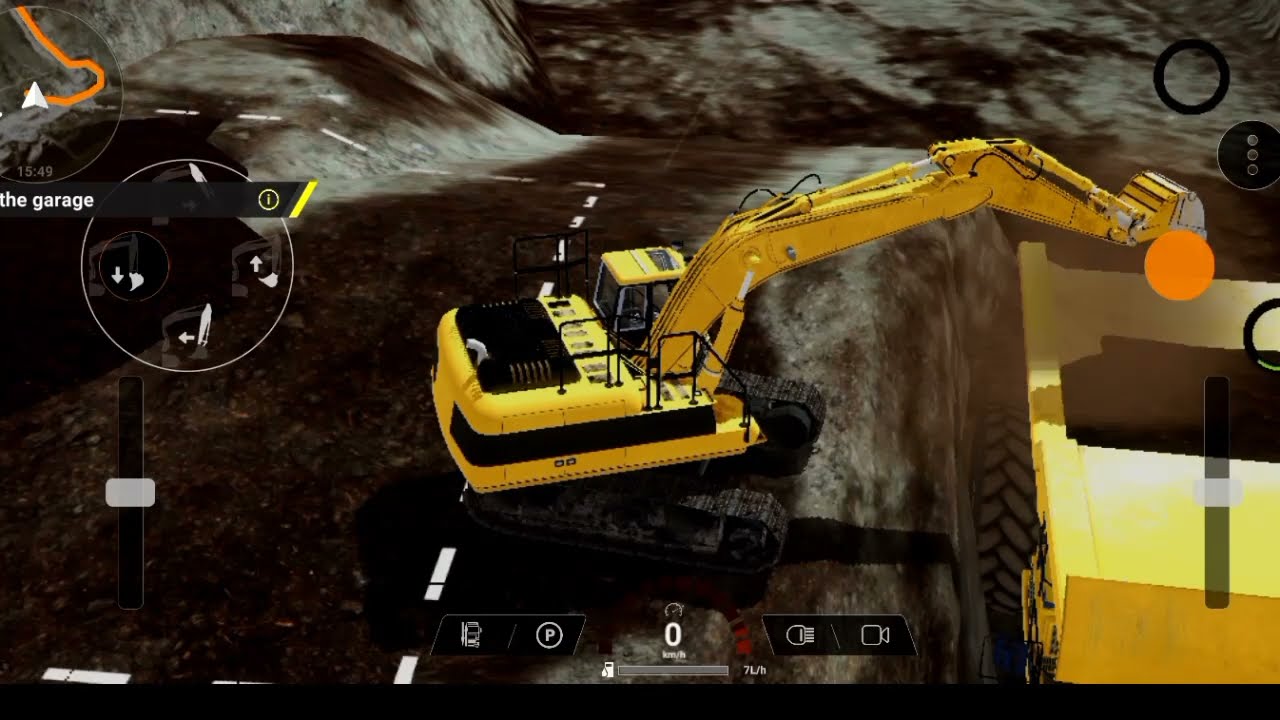This is a screenshot from a video game featuring two construction vehicles prominently at the center. The primary vehicle is a yellow forklift-like construction machine, which is in the action of lifting and dumping dirt or gravel into a second construction vehicle. This secondary vehicle, positioned to the right, is yellow with black stripes and features a truck bed filled with dirt. The background is predominantly dark gray, resembling a road surface with white dashed lines marking lanes. 

In the upper left corner, the screen displays "The Garage" with two circular icons and additional gauges. The bottom of the screen shows a digital readout of "zero miles per hour" accompanied by several icons, including one with a 'P' inside a circle and another featuring a video camera icon. There are several circular icons scattered throughout the interface; one near the bulldozer's scoop is an orange circle, and nearby, a ring-shaped icon is slightly lower. A gray bar is also visible beneath the zero miles per hour display. 

To the right-hand side of the screen, there are two circles at the top — one being a black ring and the other containing three hollow circles that look like interactive buttons. Additionally, there's a notable yellow box at the bottom right corner of the screen. The foreground and interactive elements suggest this is a digital image, likely depicting the control interface of the game.